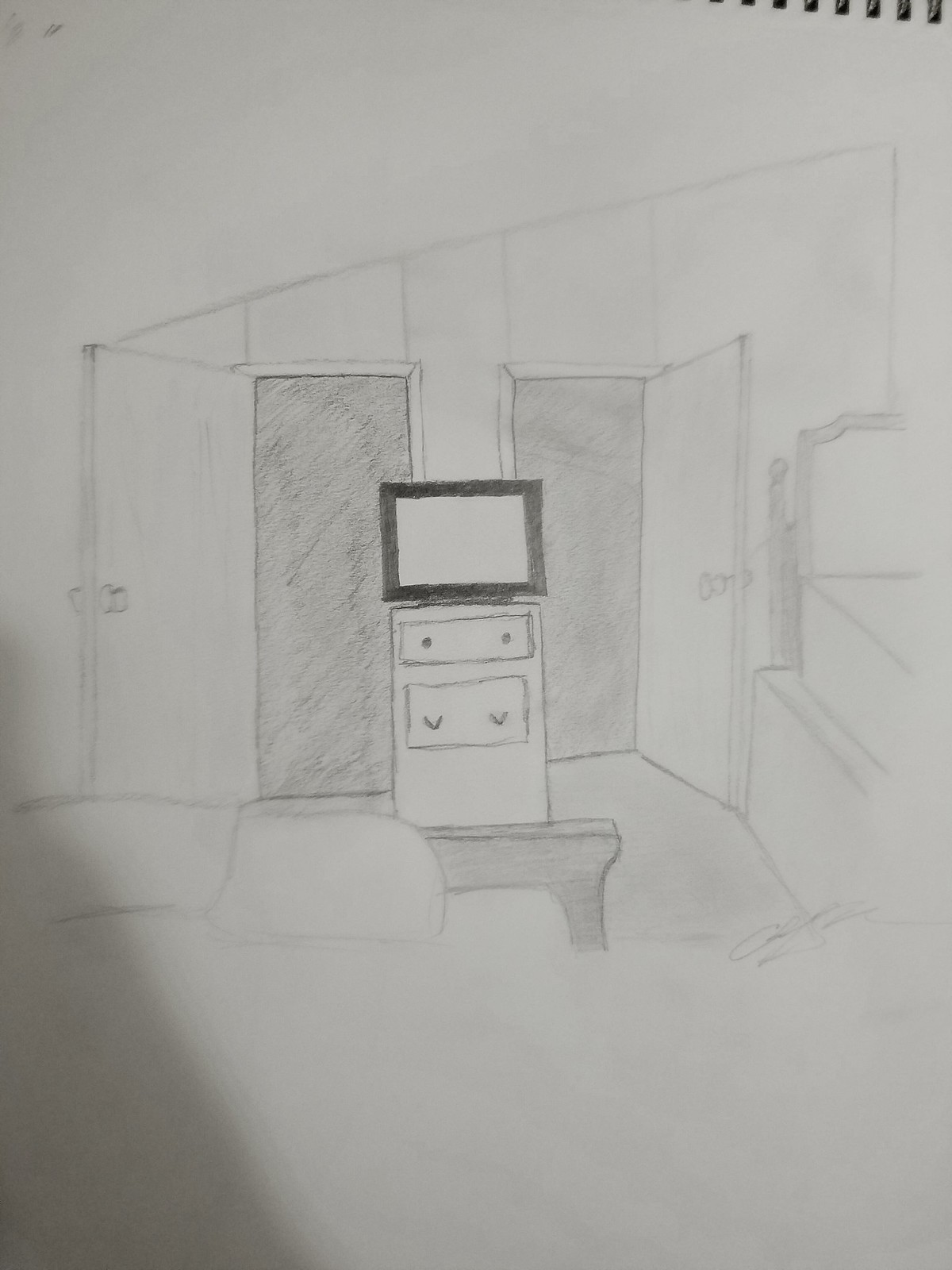The sketch is drawn on a white piece of paper from a coil-style notebook, as evidenced by the visible binder loops in the top corners. The drawing depicts a detailed bedroom scene with particular attention to perspective and shading. Centrally, there are two open doors revealing dark, shaded interiors, signifying hallways. The left door swings open to the left and the right door opens to the right. Between these doors, there is a tall piece of furniture which appears to be a combination of drawers and a cabinet. The top drawer is skinnier with two small dots as handles, and the larger bottom drawer features U-hook handles. A TV, outlined in black with a white screen, sits atop this piece of furniture.

At the front of the image, part of a bed or rug is visible, featuring what seems like a brown leg and a pillow beside it. The right side of the drawing shows another piece of furniture, possibly a higher elevated bed or bunk bed, with a distinct frame for the mattress and a box underneath. The wall behind the doors and furniture is white, adorned with vertical lines that rise diagonally towards the upper right corner, adding an element of depth.